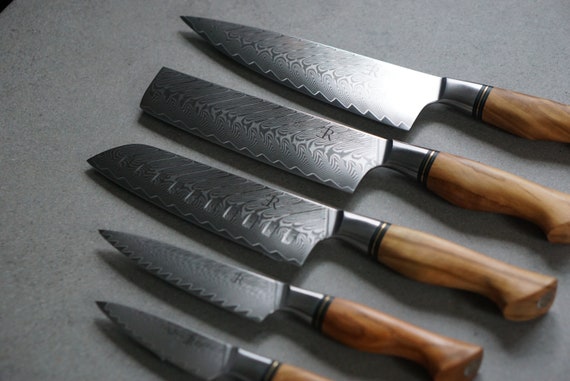This photograph showcases a detailed collection of five knives arranged in a vertical, stacked fashion on a gray stone countertop. Each knife varies in shape and size, including two small paring knives, a large chef's knife with a classic silhouette, a cleaver with a rectangular blade, and a meat-cutting knife featuring a curved blade transitioning into a squared tip. The blades are crafted with a distinctive folded steel appearance, showcasing intricate swirls and patterns that contrast light and dark areas. Notably, one blade bears a signature marked with an "R," likely the mark of the bladesmith. All knives sport elegant wooden handles with two lines delineating the handle from the blade. The image is in black and white, highlighting the unique light reflections on each blade, from a bright beam on the top knife to a darker, more contrasted middle knife. This high-definition close-up takes up most of the frame, emphasizing the craftsmanship and detail of each knife.